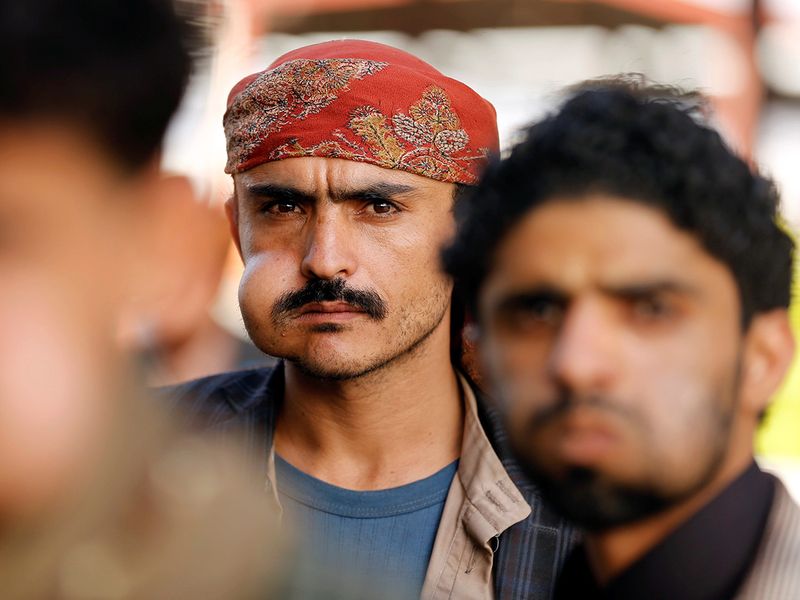The photograph captures a candid scene at a cultural event, featuring three or four male individuals of non-Caucasian descent. The focus is sharply on a central figure who is slightly left of center in the image. This man is looking directly at the camera with a furrowed brow, giving a frustrated or angry expression. He sports a black mustache and a noticeable bulge in his right cheek, suggesting he is holding something in his mouth, likely a part of the cultural event. He is adorned in a red bandana or cap with intricate filigree and embroidery along the rim, and wears a blue plaid jacket over a blue shirt. The image is framed by two out-of-focus heads in the foreground. To the left, there is a person with black hair, while to the right, another man with black curly hair, a beard, and a mustache is partially visible. This man wears a dark or dark gray shirt under a lighter-colored jacket. The background is hazy, revealing just a hint of white and pink colors, adding to the candid and spontaneous nature of the photograph.